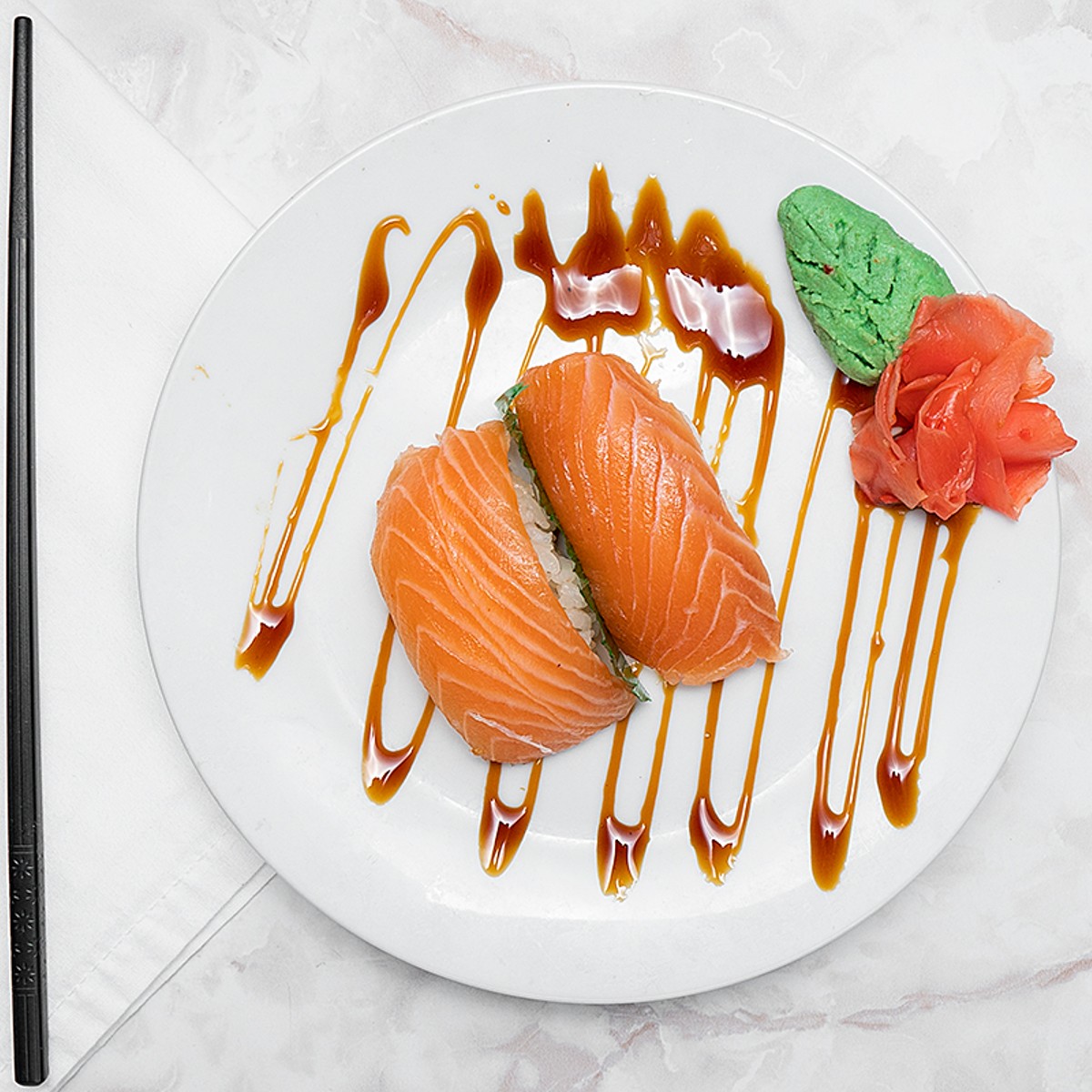The image displays a sophisticated presentation of sushi featuring a pristine white oval plate as its centerpiece. The dish includes two individual pieces of sushi, each topped with what appears to be slabs of orange tuna, with some rice slightly visible underneath. Adding to the artistic arrangement is a medium-brown sauce, carefully drizzled in a zig-zag pattern across the plate. On the right side of the plate lies a decorative clump of pink pickled ginger, artfully shaped like a flower, with a green portion of wasabi carved to resemble a leaf beside it. The setting is further enhanced by a black chopstick resting atop a neatly folded white cloth napkin positioned at the plate's edge. The entire scene is set against a luxurious white granite or marble surface, accentuating the elegant culinary presentation.